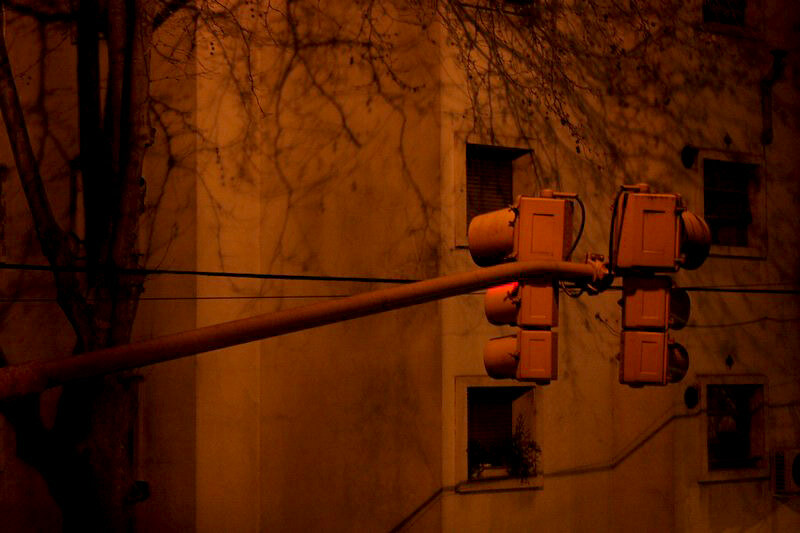The photograph captures a warm, reddish-orange tinted scene of a relatively quiet town intersection, dominated by a traffic light pole that stretches horizontally across the frame. This metal pole, appearing bare but difficult to discern precisely due to the ambient light, supports two traffic light units. Each unit houses the typical trio of red, yellow, and green lights, though the image only reveals the sides and housings of these signals, making their specific colors indiscernible. Positioned prominently in the right half of the picture, these traffic lights face opposite directions, left and right.

In the background stands a multi-story stone building, with square windows framed by deep sills. One window is adorned with plants, and another is covered with mini blinds, while the remaining windows are too shadowed to detail. Adding to the composition, a tall, leafless tree with a thin trunk casts the intricate shadows of its branches against the building’s facade, contributing to the scene's eerie warmth.